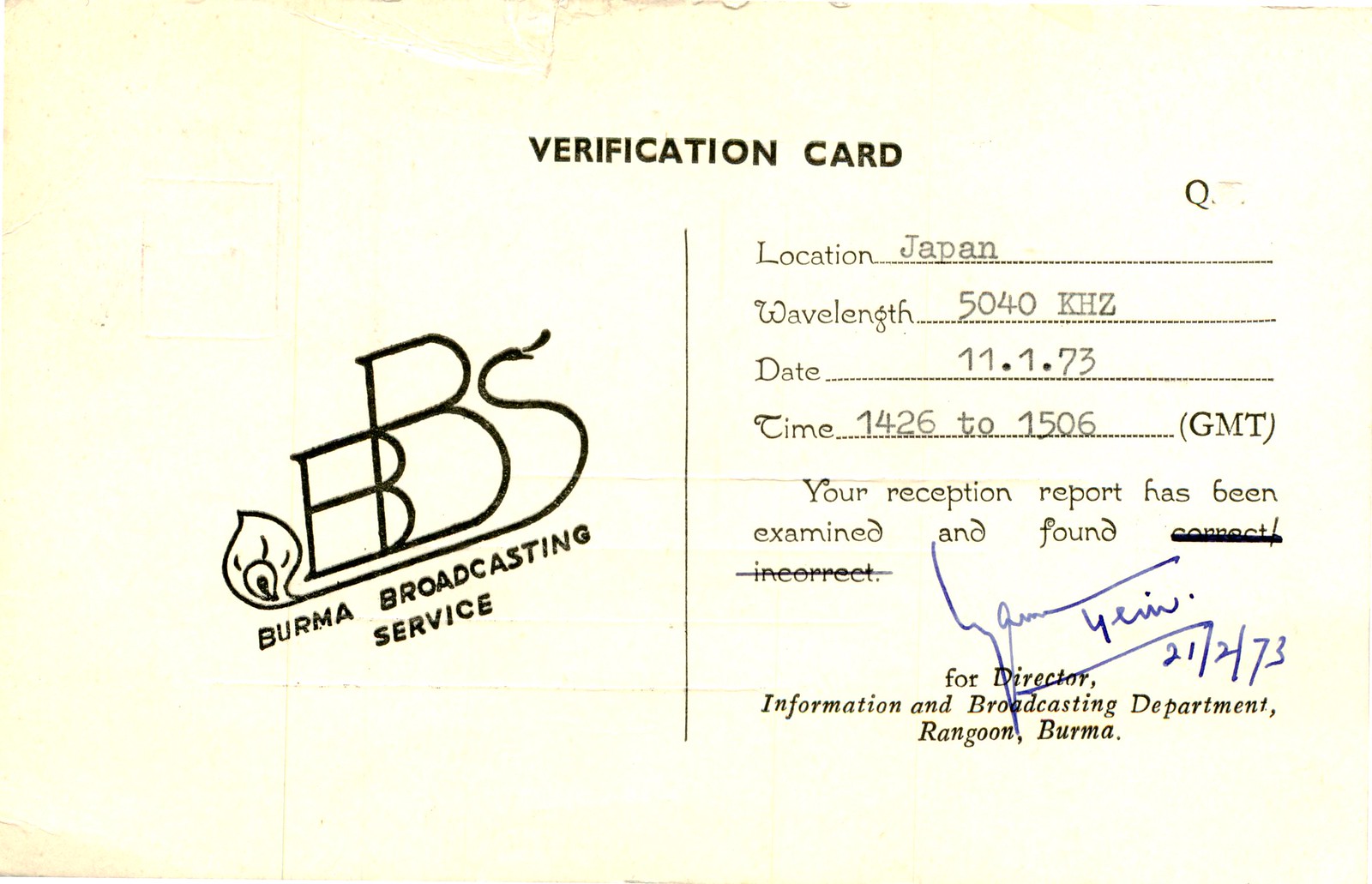This wide, vintage postcard-like verification card is made from a yellowish white paper, showing signs of aging with brown stains on the left side and at the top. The top of the card prominently features "VERIFICATION CARD" in bold black, all-capital letters. On the left side, there is a diagonal logo consisting of two large capital B's and an S-shaped snake, with "Burma Broadcasting Service" written underneath. The right side contains information typed out in black text using a typewriter: "LOCATION: Japan, WAVELENGTH: 5040KHZ, DATE: 11.1.73, TIME: 14.26 to 15.06 GMT." Below this, it reads, "Your reception report has been examined and found." Both "CORRECT" and "INCORRECT" from the original sentence have been crossed out, likely with a black marker or pen. Towards the bottom, it states, "For Director, Information and Broadcasting Department, Rangoon, Burma." There is a visible signature in blue ink along with a handwritten date of 21-2-73.